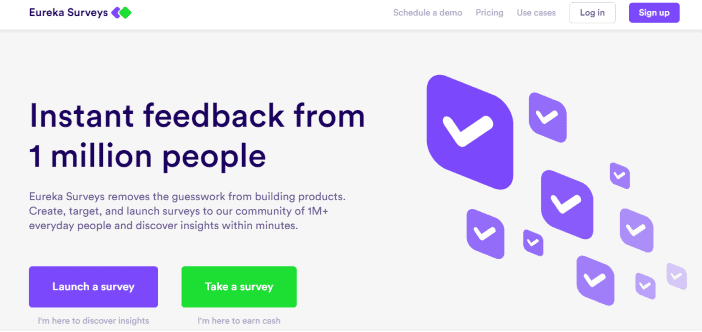The website depicted in the image is Eureka Surveys, prominently displayed in the upper left-hand corner with its logo, featuring the name "Eureka Surveys" in purple font accompanied by two overlapping diamonds—one purple and one bright neon green. On the upper right side of the page, there are navigation options including "Schedule a Demo," "Pricing," and "Use Cases," followed by two buttons labeled "Log In" and "Sign Up," with the "Sign Up" button highlighted in purple.

The primary section of the webpage has an off-white, ivory background. On the left side, a bold headline reads, "Instant feedback from 1 million people." The accompanying text explains, "Eureka Surveys removes the guesswork from building products. Create, target, and launch surveys to our community of 1 million+ everyday people and discover insights within minutes." Below this description, there are two actionable buttons: "Launch a Survey" in purple and "Take a Survey" in green.

Towards the bottom, the page offers two clear pathways for users with the phrases: "I'm here to discover insights" and "I'm here to earn cash."

To the right, the screen is decorated with multiple floating purple boxes of various sizes, each featuring white check marks. These boxes number one large and progressively smaller ones stretching from the middle left downwards to the lower right of the screen, creating a dynamic visual flow.